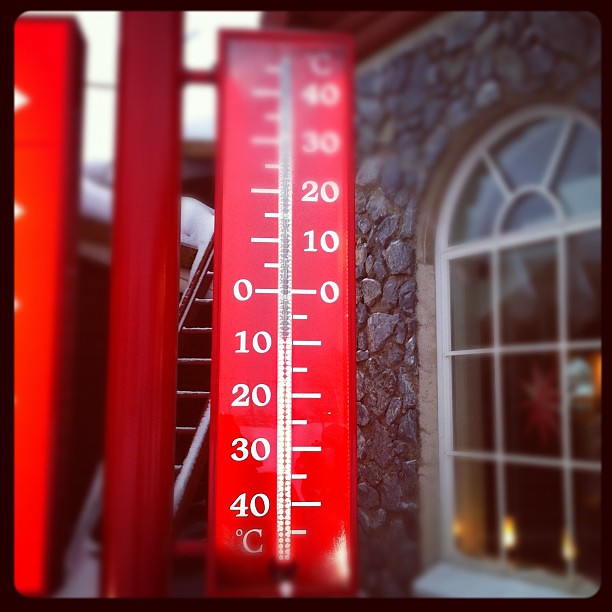This image captures a cobblestone building prominently on the right side, featuring a distinctive arched window with a grid of white mullions creating small square panes. The interior behind the window is obscured, imparting a sense of mystery about the building’s purpose—whether it be a residence or an office.

On the left side of the photo stands a large red digital thermometer displaying the current temperature in Celsius. The thermometer is designed with white numeric digits and a ruler-like measurement scale, enhancing the visibility of the temperature readout.

In the background, a staircase ascends, suggesting that this area belongs to the lower floor of a larger structure. The stairs imply an access point to a higher level, which could be another apartment, office space, or a pathway leading to the street above. The composition creates a blend of historical architecture with modern technology, offering a glimpse into an intriguing yet unclear setting.